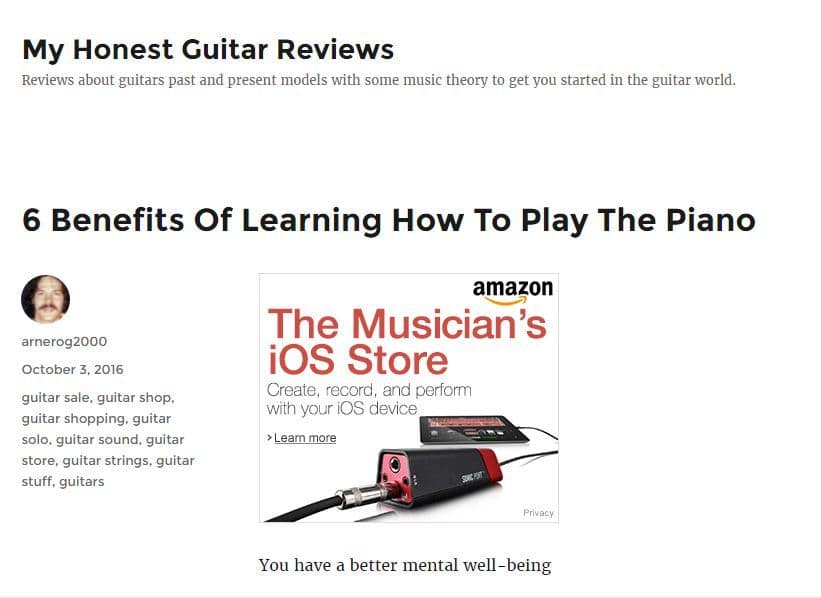In this image, we see a screenshot showcasing a detailed review on guitars. Positioned at the top left, the review is titled "My Honest Guitar Reviews," which promises insights on both past and present guitar models, along with foundational music theory tips for beginners venturing into the guitar world. Below this, there is a section titled "Six Benefits of Learning How to Play the Piano."

On the left side of the image, there's a profile icon featuring a man with a mustache, identified by the username ARNEROG2000. This review was posted on October 3rd, 2016. There is an array of tags accompanying the review, including "guitar sale," "guitar shop," "guitar shopping," "guitar solo," "guitar sound," "guitar store," "guitar strings," "guitar stuff," and simply "guitars."

To the right of the review, there's an Amazon advertisement prominently featuring the Amazon logo in the upper right corner. The ad highlights "The Musician's iOS Store," encouraging users to create, record, and perform music using their iOS devices. There's a "Learn More" button included in the ad text, with additional text beneath it stating "You have a better mental well-being."